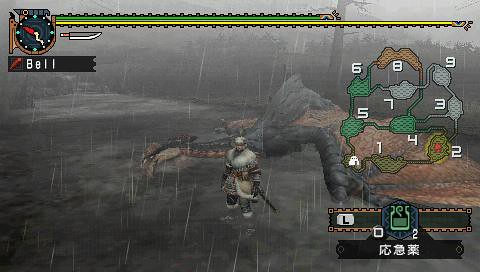In this screenshot of a video game, the scene is drenched in rain, depicted by long, thin, white shards falling from the sky. Central to the image is an armored figure, presumably a knight, adorned with medals and garb, and wielding a sword. The knight stands over a large, deceased creature, possibly a dragon, which lies in the water, displaying gray and brown hues. Above the scene stretches two bars, one green and one yellow, likely indicating the player's health. On the top left, the character's name, "Bell," is displayed alongside a circular compass marked with a red directional arrow, and a depiction of a sword with a brown handle and a gray blade. A map is visible on the right, highlighted with the numbers 1 through 9 in white, and shows various terrains in green, brown, and gray. The overall color scheme of the image is dominated by grays and browns, adding to the somber and moody atmosphere.